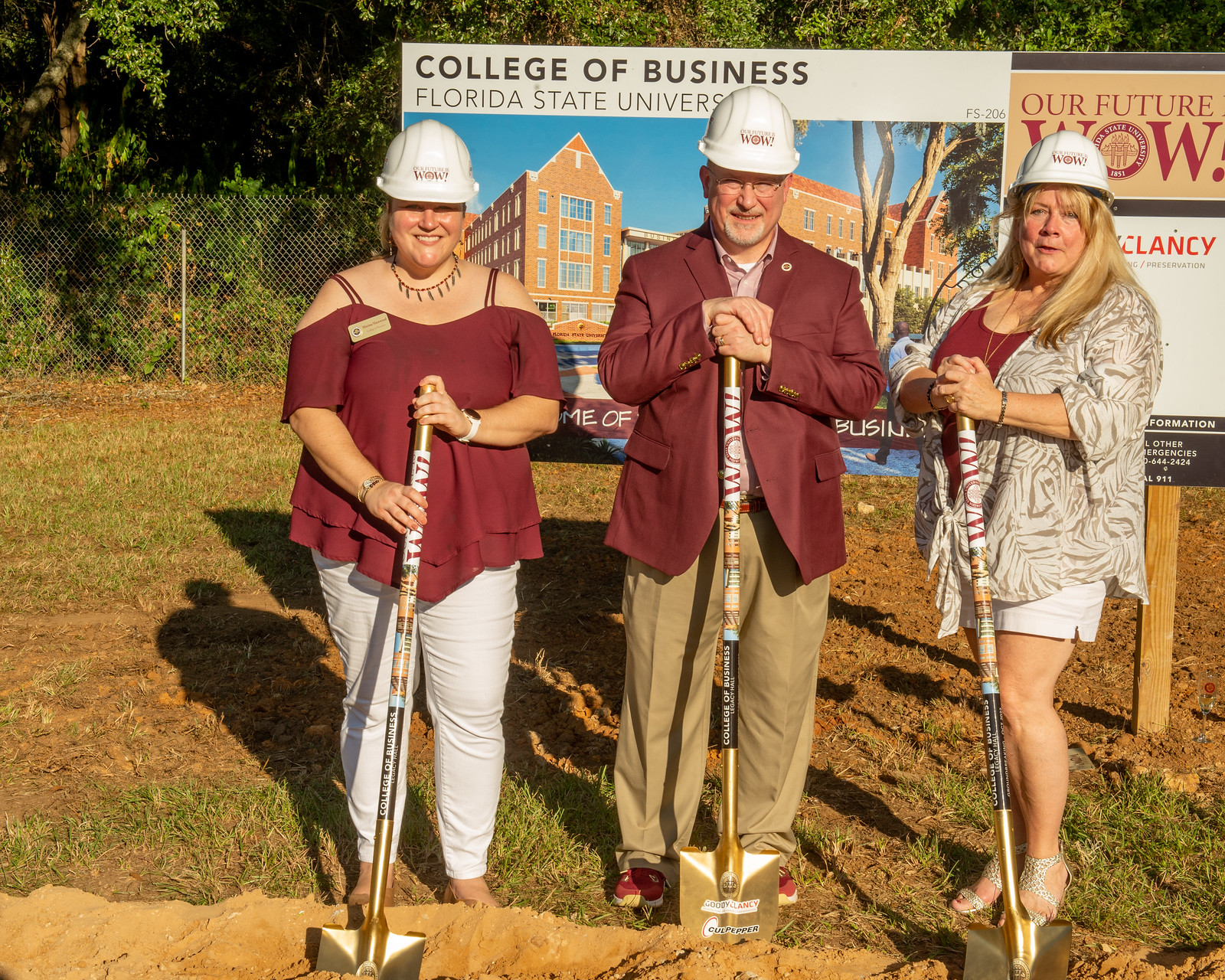The image captures a groundbreaking ceremony for the College of Business at Florida State University. Three individuals, likely faculty or administrators, are all smiles as they commemorate the start of construction on a new building. Each person is equipped with a golden shovel, emblazoned with “WOW” – a slogan that appears on their white construction helmets as well, where the “O” features the school's logo. Despite the formality of their attire, which includes a woman in a red shirt and white pants, another woman in shorts, and a man in a red jacket and suit, they are joyously celebrating the occasion. The backdrop includes a detailed architectural plan showcasing a traditional, four-story brick building, reinforcing their significant accomplishment.